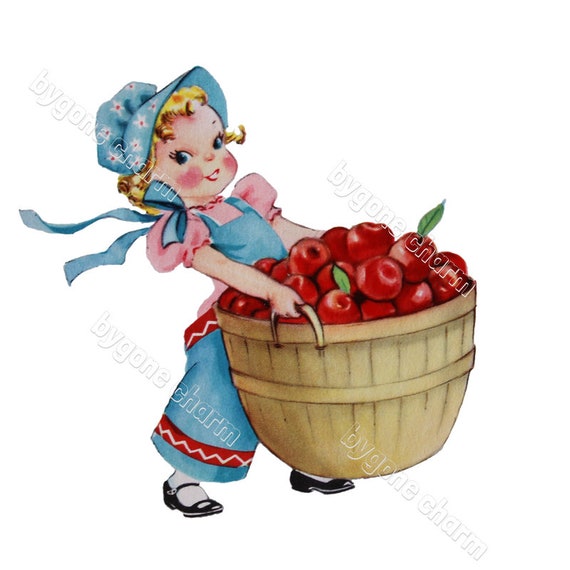The drawing depicts an old-fashioned cartoon rendering of a little girl with blonde hair, wearing a blue-flowered bonnet tied at the side of her neck, a blue ribbon that matches her blue eyes and rosy cheeks. She sports a pink shirt under blue overalls adorned with red accents and a white zigzag pattern. On her feet, she has black shoes with straps and white stockings. The girl is carrying an oversized wooden wicker basket, structured with two circular frames enclosing the vertical slats, filled with bright red apples, two of which have single leaves. Despite the basket appearing heavier than she is, she smiles as she moves from left to right across the image. The drawing features repeated watermarks reading "Bygone Charm," that fade across the image, reinforcing a nostalgic charm.